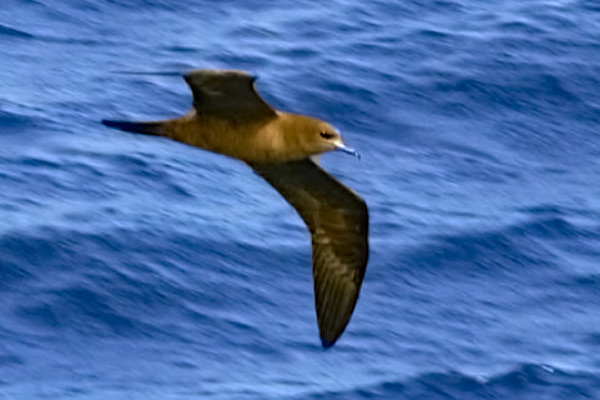The image captures an action shot of a sleek, brown water bird soaring over a textured, graphic background depicting a vibrant blue body of water with waves and ripples. The bird, facing the right-hand side of the frame, has outstretched dark brown wings that taper to pointed ends, resembling a boomerang in shape. Its body is streamlined and cigar-shaped with a tannish-brown hue, and it features a straight tail and a long, dark beak with a slight hook at the tip. Despite the slight blur indicating the bird's swift movement, one can see its intense, dark eyes as it appears to be searching for prey below. The backdrop showcases contrasting shades of blue, accentuating the sense of motion and the bird's high-speed flight over an almost illustrative rendition of the ocean.